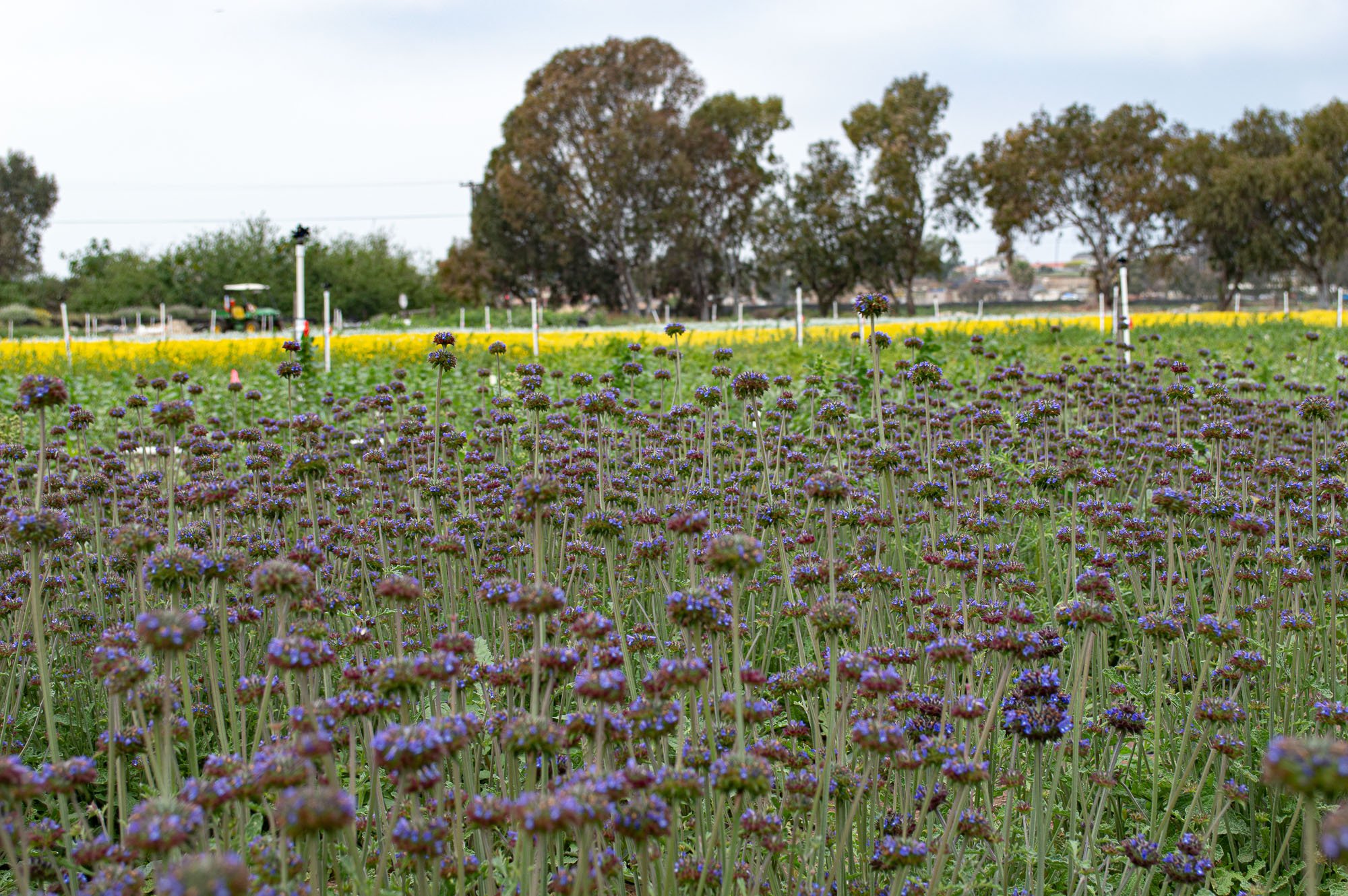This landscape-oriented image captures a serene, vibrant field predominantly filled with delicate, small purple flowers. These flowers, with their tiny petals forming near-bulbous clusters, are scattered throughout the expansive green grass. The photo is taken at flower level, emphasizing the rich purple hues contrasting with the lush greenery. Amongst the purple flora, occasional yellow flowers add a bright splash of color to the scene.

The field extends into a secondary layer of primarily yellow flowers in the midground. Beyond this, a line of trees, comprising mostly green-leafed and some brown-leafed specimens, borders the background. In this hazy distance, a green tractor with a white canopy is discernible, hinting that this area might be part of a farm. Behind the tractor, a blurred cityscape with visible buildings adds depth to the scenery. The sky overhead is a mix of light blue, accented by wisps of white clouds, completing this picturesque outdoor setting.